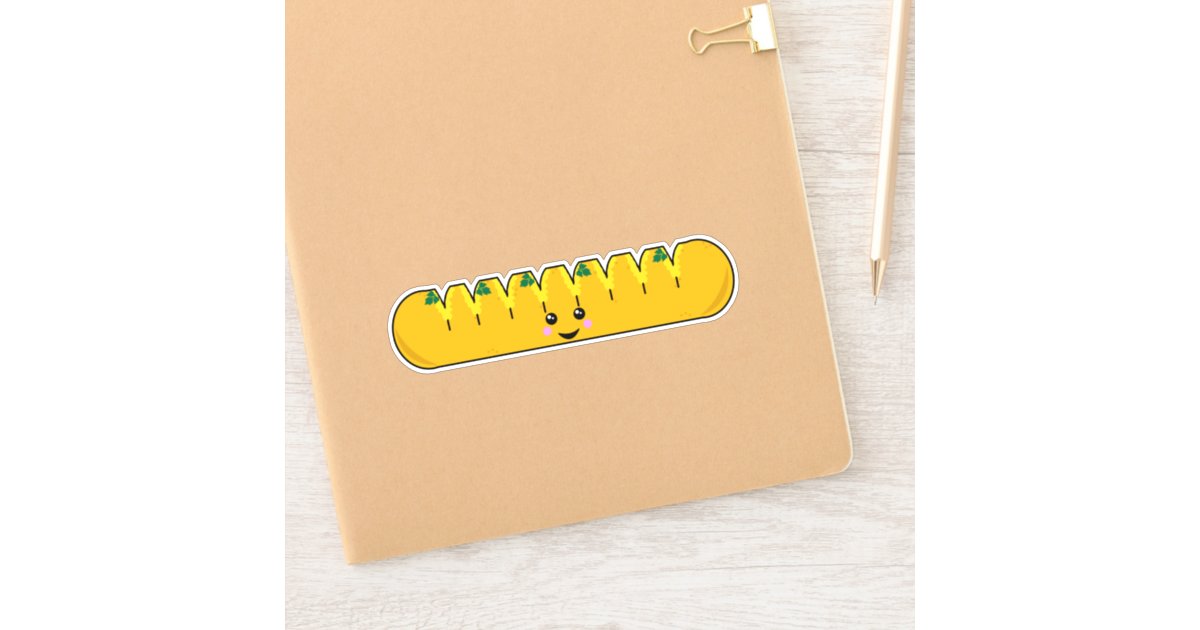The image features a beige folder positioned at an angle from the left. The background showcases a blonde wood surface, potentially a table. The folder is adorned with a cute, cartoon drawing of a yellow, pill-shaped cartoon character resembling a loaf of garlic bread or a smiling baguette. This cartoon bread has green accents at the top and is characterized by several ridges that might represent cuts in the bread. It sports black eyes and a cheerful, upward-curved smile, with pink circular marks indicating blushing cheeks. A white binder clip with gold-colored metal secures the top right corner of the folder. Additionally, a white pen lies on the wood surface in the upper right-hand corner of the image.